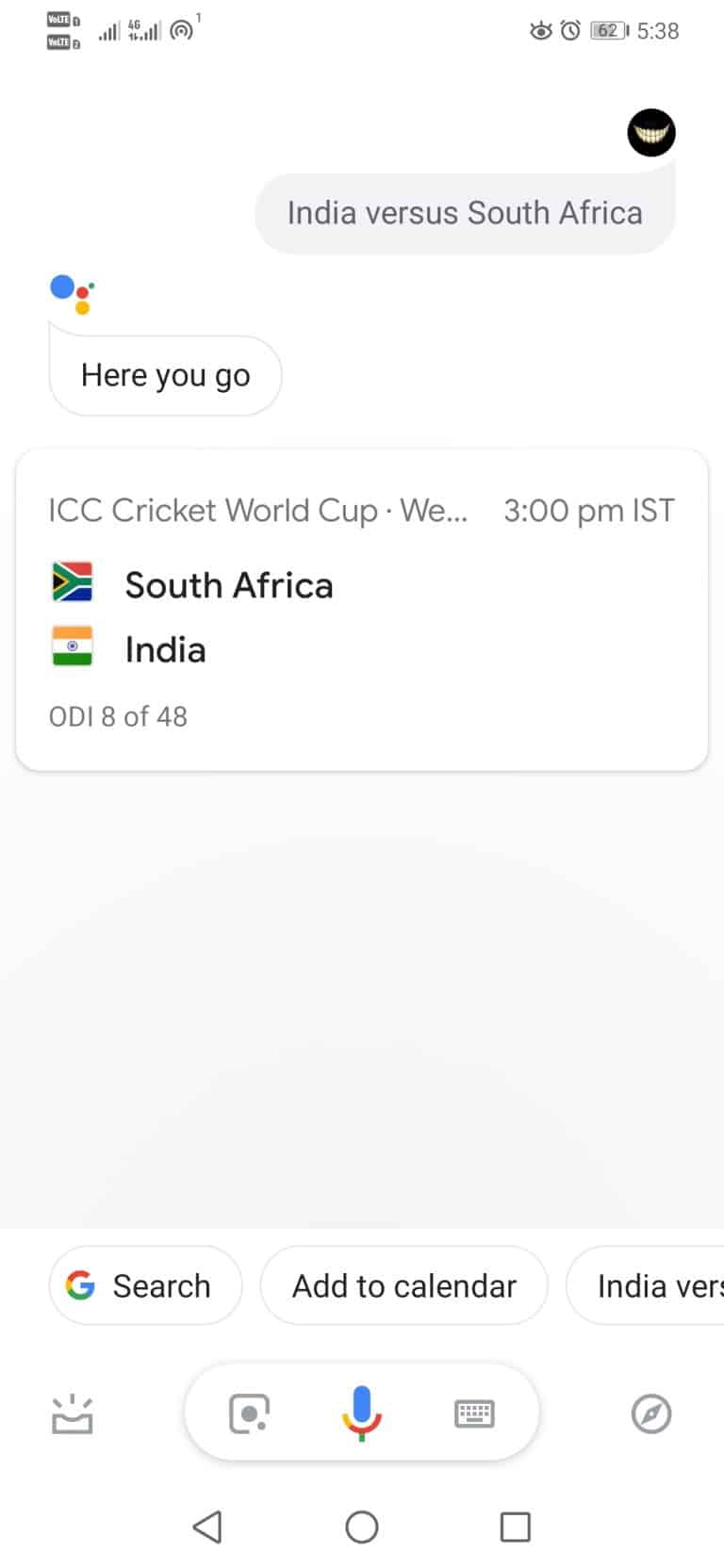Here's a detailed and cleaned-up caption for the image described:

---

The screenshot captures a Google Assistant interface, believed to be from Google Bard before its rebranding to Gemini. The background is predominantly white. At the top, the phone’s status bar shows the time as 5:38 PM with a 62% battery charge. In the upper right corner, a light gray box with gray font indicates the search prompt "India versus South Africa."

Below this prompt, the Bard icon from the Google Bard phase is visible. This icon is a blue circle with a smaller red circle atop a smaller yellow circle. The text "Here you go" follows the icon, leading into the match details:

- **Event:** ICC Cricket World Cup
- **Time:** 3 p.m. IST
- **Teams:**
  - **South Africa:** The country's flag appears to the left of its name.
  - **India:** The Indian flag is shown to the left of its name.

The interface features ample white space below the match information. At the bottom part of the screenshot, the footer includes:
- On the left, the Google "G" logo in its characteristic red, yellow, green, and blue colors, with the word "Search" beside it.
- In the center, the option "Add to calendar."
- On the far right, the beginning of the word "India," followed by "BER," presumably the start of a truncated word.

Towards the bottom center, a blue microphone icon is displayed. To the left of this, there is an icon likely representing Google Lens, and to the right, an icon for the keyboard. At the very bottom, there are three navigation icons: a gray outlined square, a gray triangle pointing left, and another icon which is not detailed in the provided description.

---